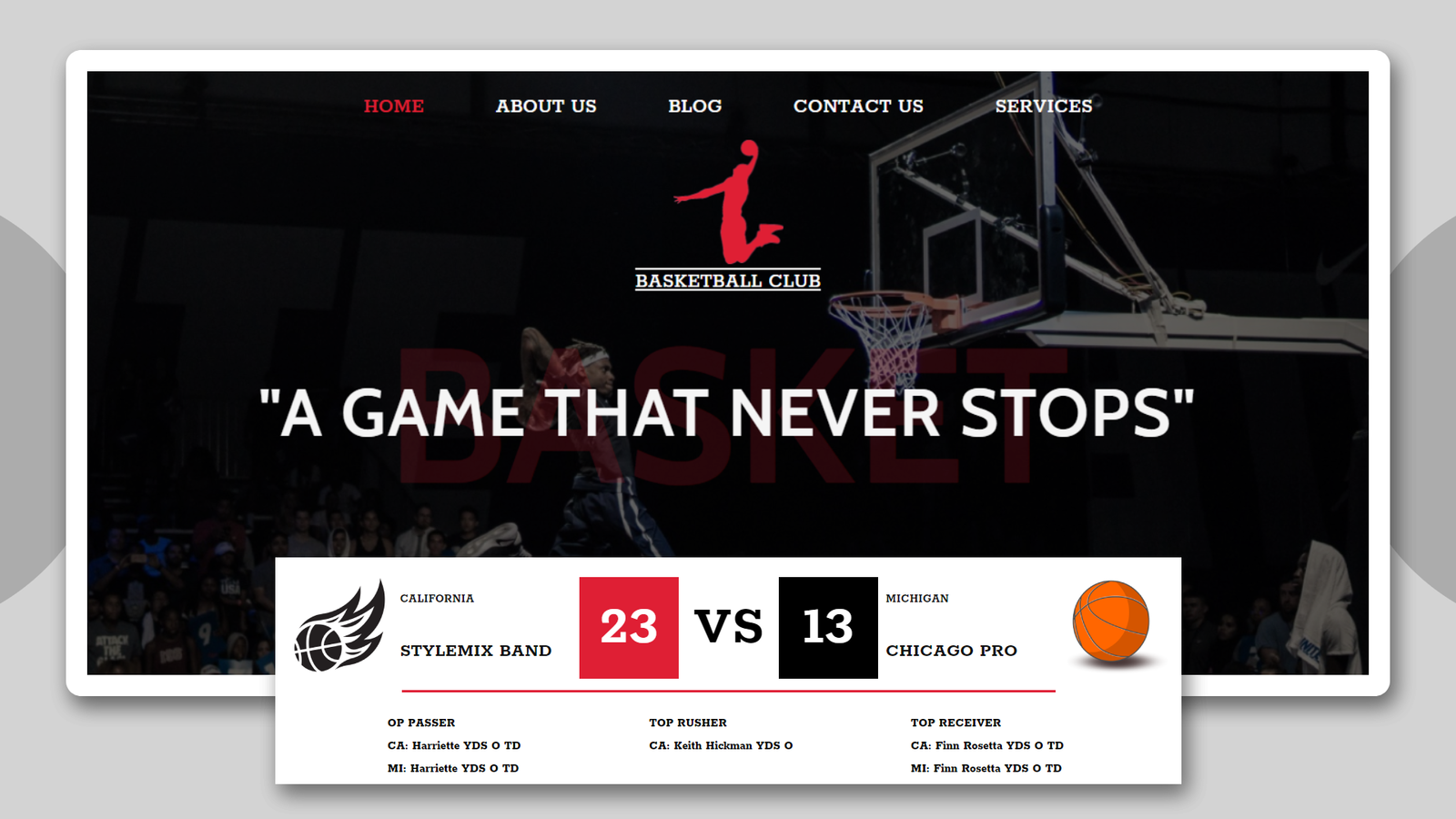The image features a multifaceted design set against a primarily light gray background. Notably, two-thirds of a circle appear on both the left and right sides, contributing to the composition’s symmetry. The main image itself is framed with a white border against a very dark backdrop. 

In the upper right area of the dark background, there is a basketball hoop. To the left, a player is depicted mid-air, reaching up to dunk a basketball. 

At the center top of the image, there is a dynamic red silhouette showing a figure holding a basketball in their right hand, knees bent, shoes up against their backside, poised for a dunk. Directly below this silhouette, a white line precedes the text "BASKETBALL CLUB" in capitalized, Georgia-style font. This is followed by another white line, all centered and justified for visual alignment.

Situated at the top of the frame is a menu bar. The menu options are predominantly in white, with the exception of the "HOME" option on the far left, highlighted in red to denote its selection status. The remaining menu options, 'ABOUT US', 'BLOG', 'CONTACT', and 'SERVICES', are in white.

Beneath the logo, a quote in large white text reads, "A GAME THAT NEVER STOPS."

At the bottom of the image, a central overlay attracts attention. To the left within this overlay, a basketball with flames shooting from its top right corner is depicted. Directly above this, in small black capital letters, it reads "CALIFORNIA," and below, in larger but similar font, it states "STYLE MIX BAND." 

To the right of this fiery basketball depiction, a red square with the white number "23" stands out, followed by "VS" in black letters, and then a black square with the white number "13," indicating a score between two competing teams.